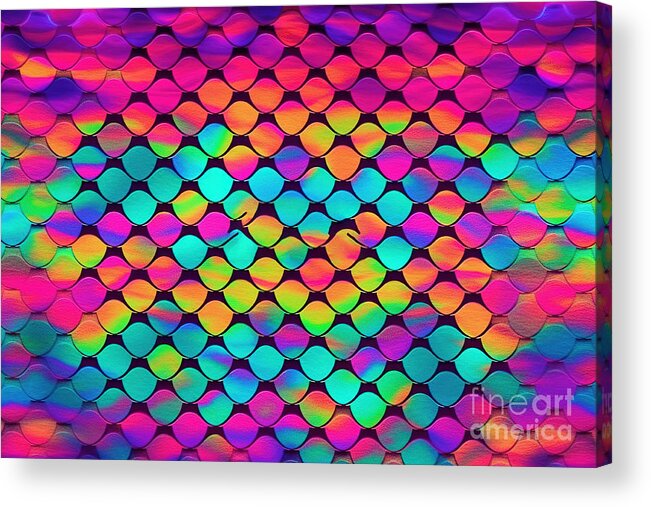This artwork, digitally rendered and titled by "Fine Art America" in faded letters at the bottom right, evokes the nostalgic imagery of the beloved "Rainbow Fish" storybook. Dominating the entire canvas, a geometric pattern of fish-scale-like circles fills the space with vivid hues and a sense of motion. Each scale-like shape aligns in a precise grid, angling at 45 degrees, reminiscent of vertically stacked eggs, creating an intricate and orderly arrangement. The palette bursts with vibrant, almost neon colors, including shades of bright aqua, orange, pink, yellow, lime green, and deep purples, reflecting a rainbow wash that intensifies toward the metallic-like center, giving it an eye-catching sheen. This multifaceted and brilliant piece captures the essence of a rainbow, transforming it into a mesmerizing and structured visual symphony.